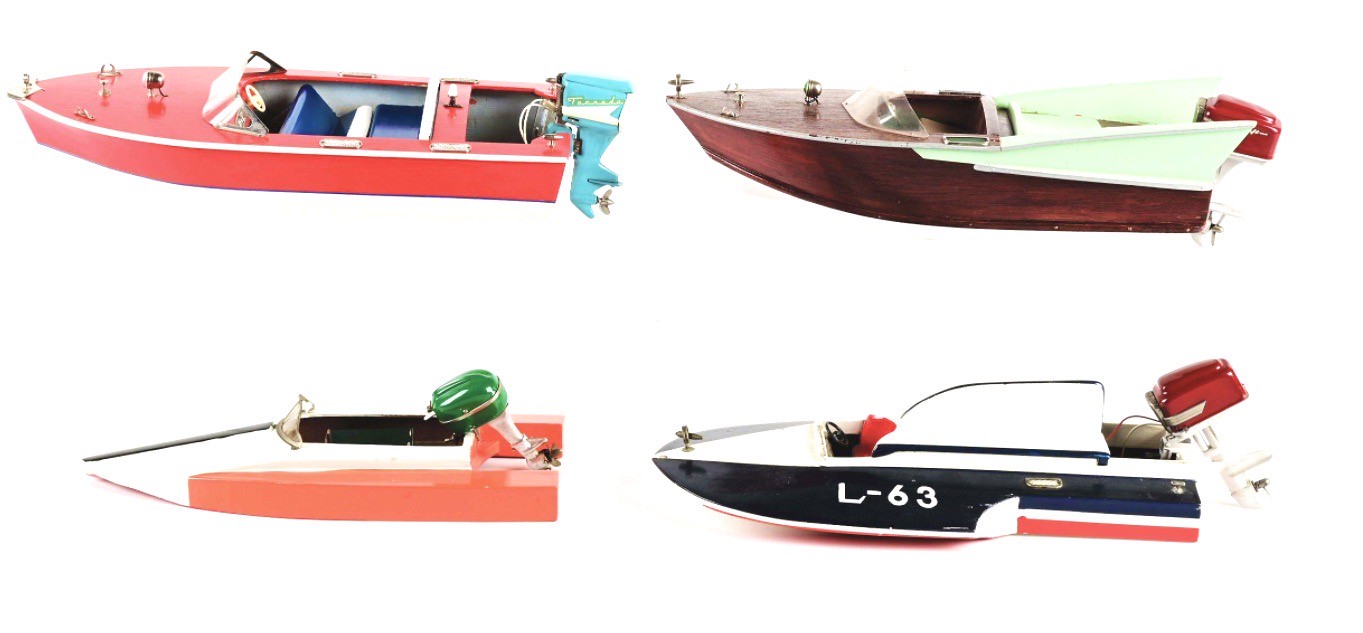This illustration depicts four meticulously detailed miniature speed boats, all facing left, seemingly driving in that direction, set against a crisp white backdrop. Starting from the upper left corner, the first boat is primarily reddish with a white trim running along its side. It features a glass dome over the yellow steering wheel, blue and white seats, and a distinctive teal-blue motor hanging off the back. Directly to the right of this boat is a natural wood boat accented with mint-green fins on each side. It houses brown seats and a red motor extending downward.

Moving to the lower section, the boat on the left is noticeably smaller, characterized by its peachy-red hue with white at the hull. This boat sports green upholstered seating and a matching green motor. Finally, in the lower right corner, the fourth boat stands out with its deep navy blue color, complemented by white and red stripes and the inscription "L-63" in white on its black section. The seats are not clearly described, but it features a prominent red motor with a lower white portion. These boats, crafted with great attention to detail, capture a blend of vibrant colors and unique features, showcasing the intricate artistry involved in their creation.